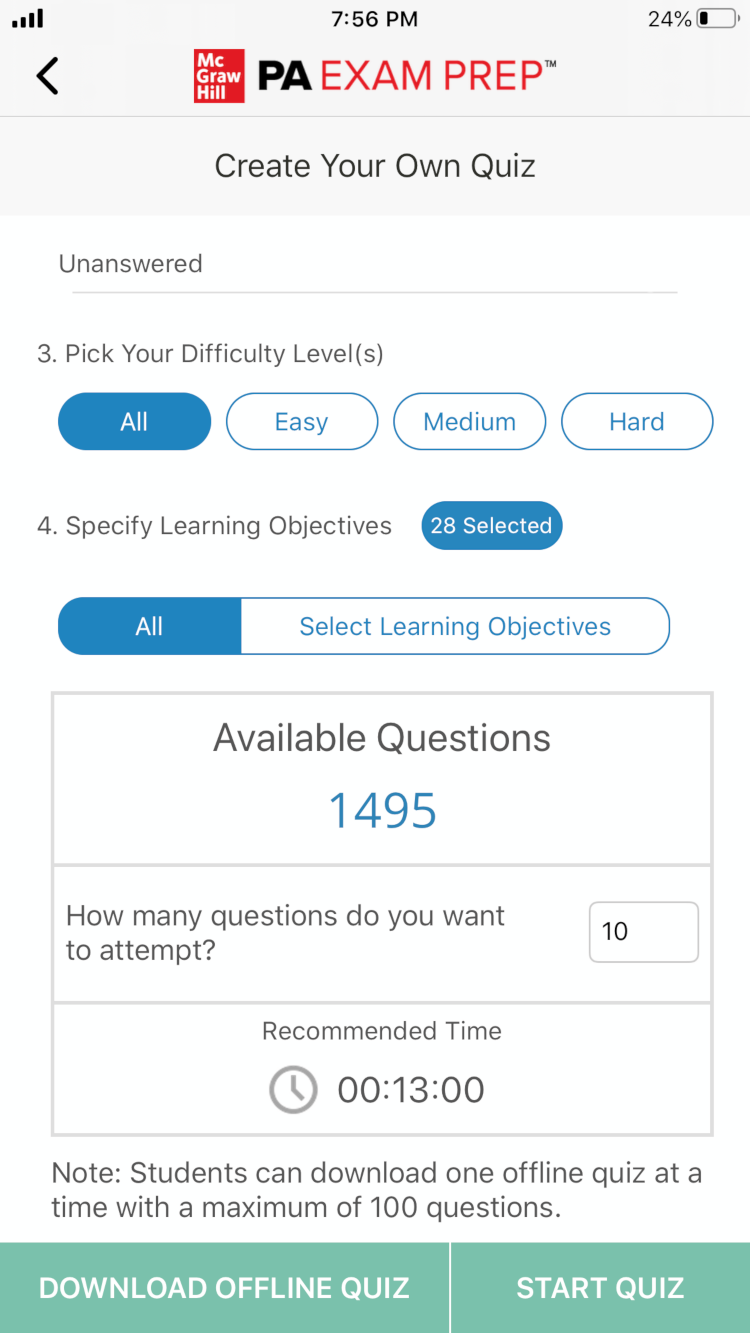Screenshot Description:

The screenshot displays a user interface on a white background with several elements and options, providing users the ability to create their own quiz.

- At the top, there is a status bar displaying the time "7:56 PM" and the battery percentage "24%".
- Below, there is a red square containing the name "Matt Grawhill" in white text, with a left-pointing arrow next to it.
- The main content area is titled "PA Exam Prep".
- Below the title, there is a section labeled "Create Your Own Quiz" with the status "Unanswered".
- Users are prompted to "Pick your difficulty levels," with four ovals to choose from: "All," "Easy," "Medium," and "Hard."
- There are four specified learning objectives listed. One blue oval shows "28 selected," and another blue oval labeled "All." Additionally, there is a white oval for selecting learning objectives.
- The interface lists "Available Questions" with a count of "1,495."
- Users can specify "How many questions do you want to attempt," with a default number of "10" set.
- The recommended time for completion is indicated by a clock icon showing "00:13:00".
- A note indicates, "Students can download one offline quiz at a time with a maximum of 100 questions."
- At the bottom, there is a blue rectangular button labeled "Download Offline Quiz."

This detailed description highlights the user interface elements and options available for creating and downloading a personalized quiz.